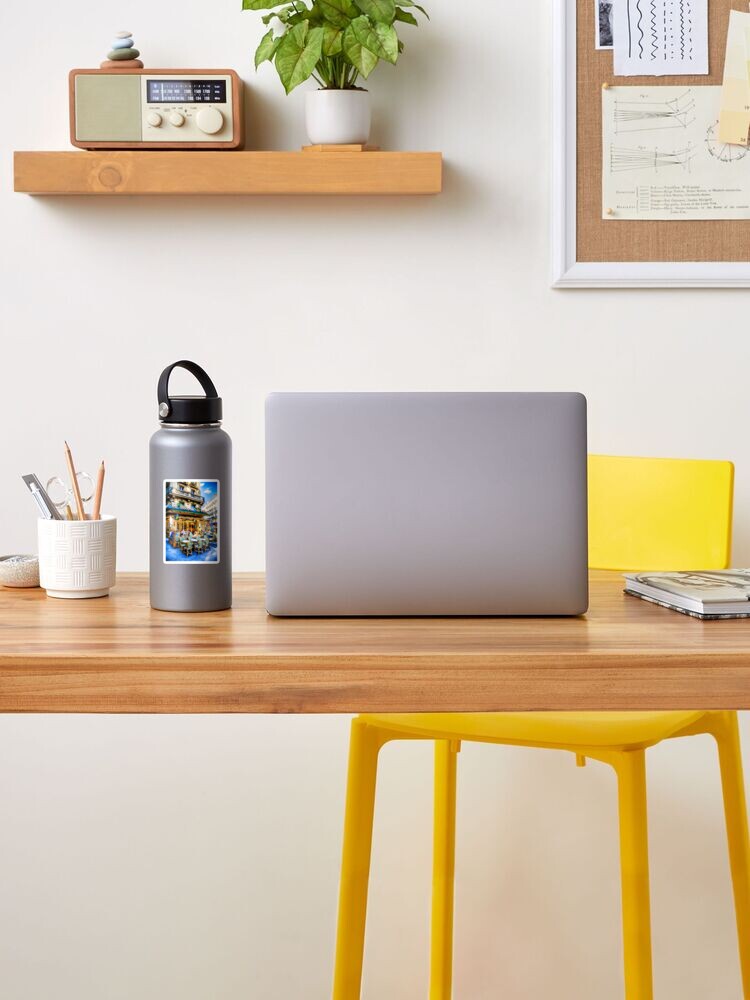This photograph depicts a well-organized home office setting. The focal point is an oak-colored wooden desk with a sleek silver laptop placed centrally. To the left of the laptop sits a gray metal water bottle, decorated with a city-themed sticker, and further left is a white ceramic cup holding two pencils, a pen, and a pair of scissors. A book also lies on the desk. Positioned behind the desk is a distinctive yellow chair with four legs.

The office's back wall is painted a bright white, creating a clean and inviting atmosphere. Attached to the wall, above the desk, is a floating oak-colored wooden shelf. The shelf displays a small potted plant in a white planter and a vintage 1970s-style radio with a wood grain frame, which is adorned with a couple of colorful rocks.

To the upper right of the photo, a corkboard is visible. This board has several papers pinned to it, including graphs and other documents. The entire setup conveys an efficient and aesthetically pleasing workspace.